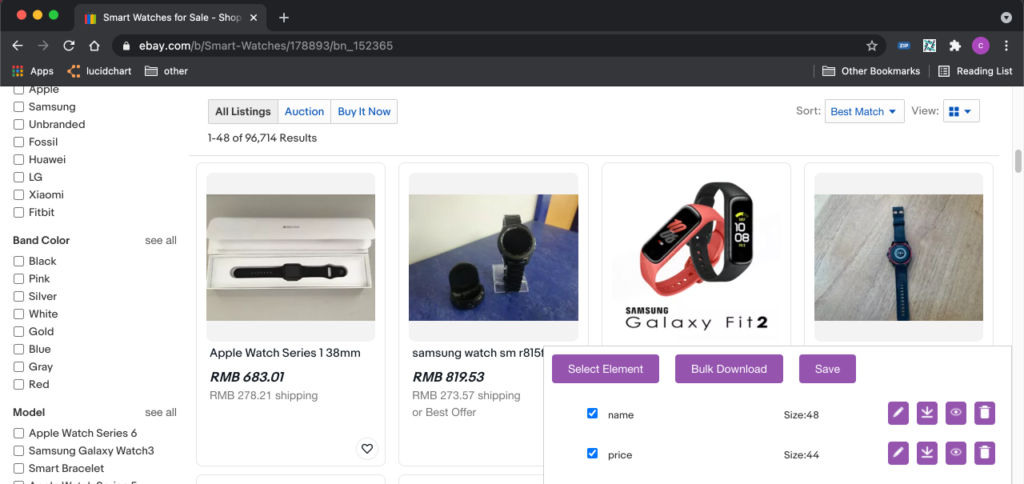This image is a screenshot of a user's eBay browsing session in night mode. The browser window features a dark gray top bar, typical of night mode settings, with the familiar red, yellow, and green buttons on the top left for expanding, minimizing, or closing the window. The open tab is labeled "Smartwatches for Sale," accompanied by the eBay logo, indicating the user is on the eBay website.

At the top center of the screen, a search bar shows the URL "ebay.com/smartwatches," confirming the specific section of the website being browsed. Below the search bar, there are bookmarks and quick links to apps and tools such as Lucidchart, greeting lists, and profile options.

On the right side of the page, there is a column dedicated to refining search results, allowing the user to filter smartwatches by brand, color, and model. Adjacent to this column, the main content area displays various smartwatch listings, each featuring discounted prices and percentage savings.

Above the smartwatch listings, navigational options allow the user to toggle between "All Listings," "Auction," and "Buy It Now" formats. The search results indicate 1 out of 48 of 96,713 total results. There are four highlighted smartwatch options, each with images and basic details, and a toolbar at the bottom of this section appears with options to "Select," "Bookmark," "Download," or "Save," complete with checkboxes for selecting items by name or price.

At the very top of the smartwatch listings, there is a sorting option set to "Best Match," and the view is arranged in a grid style. On the far right of the screen, a vertical scroll bar is visible, indicating the possibility of more content below the visible area.